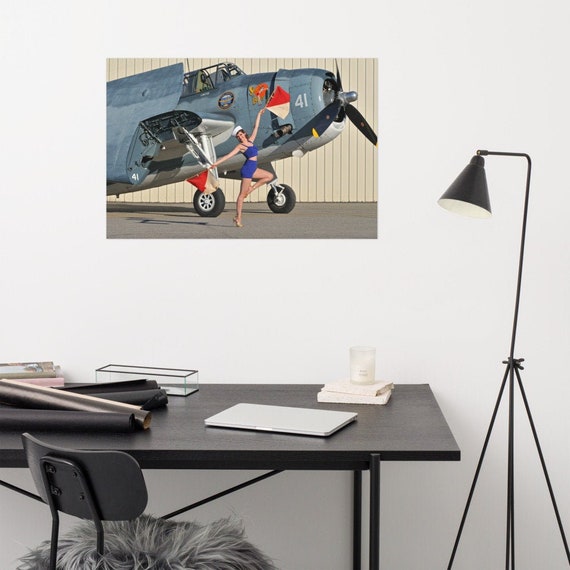The image features a sleek, black desk with a gray surface, positioned against a white wall. On the desk lies a closed laptop and several large, rolled-up black papers, potentially samples. A black chair sits in front of the desk, equipped with a plush, fluffy cushion that has long, fur-like hairs for added comfort. Adjacent to the desk is a simple floor lamp made of black cast iron, its head directed towards the desk. Dominating the white wall is a colorful, vintage-style poster of a gray airplane marked with the number 41. In front of the plane, a woman poses in a dynamic, dance-like stance. She stands on one leg, with her other knee bent and her foot resting on her supporting thigh. Dressed in a royal blue bikini and a vintage military hat, she holds red and white flags—her left arm raised high, and her right closer to the ground. The poster exudes a pin-up style, adding a lively contrast to the otherwise monochromatic room.